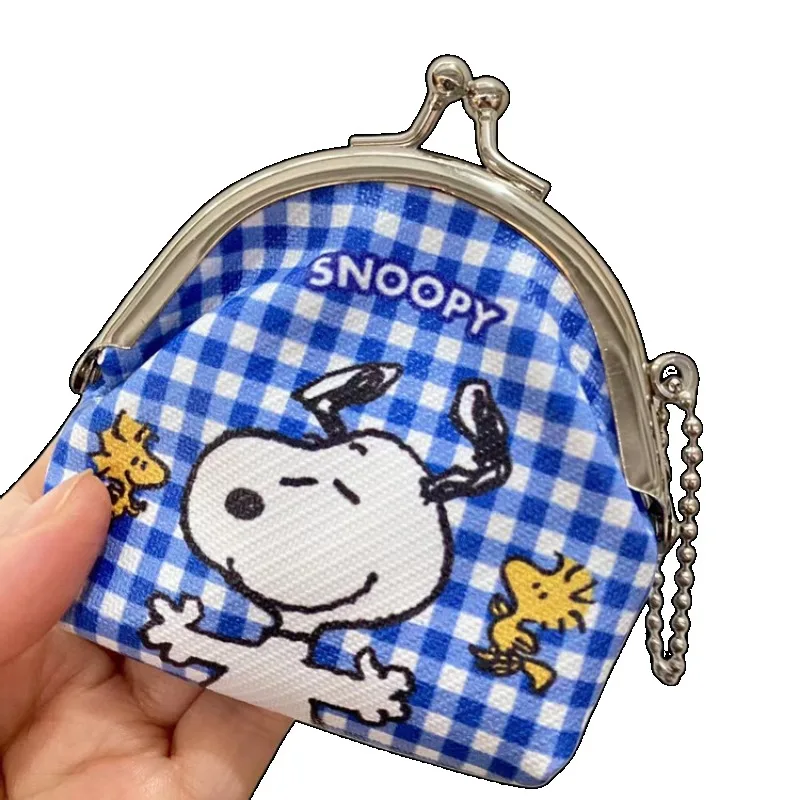In this photograph, a person is holding up a large coin purse with their left hand. The purse features a striking blue and white checked pattern, reminiscent of a tablecloth, with the word "Snoopy" prominently displayed. The iconic character Snoopy, accompanied by two small birds, is illustrated on the front. The purse is secured with a silver clasp at the top, which pops open for easy access. It also includes a small chain on the side, potentially for attaching to a belt or bag. The size of the purse appears somewhat larger than a typical coin purse, suggesting it might be used for carrying multiple items or a substantial amount of change.